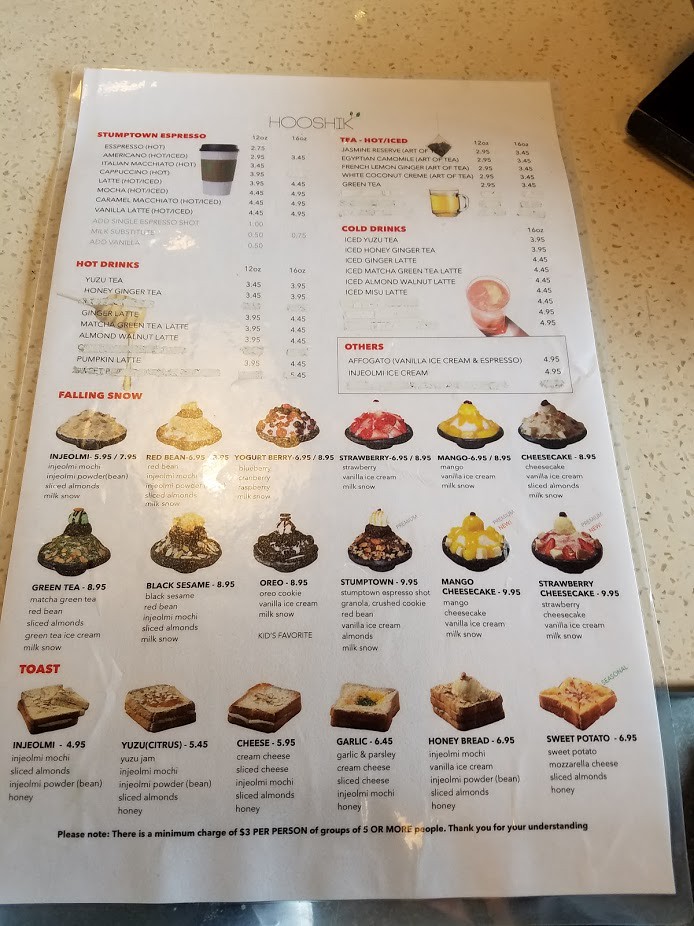The photograph captures a detailed, color image of a white laminated menu, set against a white and brown speckled surface. The menu header spells out "H-O-O-S-H-I-K." The extensive list of items includes a variety of hot and iced beverages, teas, and specialty drinks, along with their respective prices and available customizations.

The menu starts with a selection of espresso drinks from Stumptown Espresso:
- Espresso (hot, 12 oz) - $2.75
- Americano (hot/iced) - $2.95
- Italian Macchiato (hot) - $3.45
- Cappuccino (hot) - $3.95
- Latte (hot/iced) - $3.95
- Mocha (hot/iced) - $4.45
- Caramel Macchiato (hot/iced) - $4.45
- Vanilla Latte (hot/iced) - $4.45

Customers can add a single espresso shot for $1, choose a milk substitute for $0.50, or add vanilla for $0.50.

The tea section offers various flavors:
- Jasmine Reserve - $2.95
- Egyptian Chamomile - $2.95
- French Lemon Ginger - $2.95
- White Coconut Cream - $2.95
- Green Tea - $2.95

Under hot drinks:
- Yuzu Tea - $3.45
- Honey Ginger Tea - $3.45
- Ginger Latte - $3.95
- Matcha Green Tea Latte - $3.95
- Almond Walnut Latte - $3.95
- Pumpkin Latte - $3.95

For cold drinks:
- Iced Yuzu Tea - $3.95
- Iced Honey Ginger Tea - $3.95
- Iced Ginger Latte - $4.45
- Iced Matcha Green Tea Latte - $4.45
- Iced Almond Walnut Latte - $4.45
- Iced Miso Latte - $4.45

The section for other treats includes:
- Affogato (Vanilla Ice Cream and Espresso) - $4.95
- INJEOLMI Ice Cream - $4.95

Next listed are items under "Falling Snow," with accompanying photographs of dishes filled with shaved ice and various toppings:

- INJEOLMI ($5.95/$7.95) includes INJEOLMI Mochi, Powder, Beans, Sliced Almonds, and Milk Snow.
- Red Bean ($6.95/$8.95) features Red Bean Mochi, INJEOLMI Powder, Sliced Almonds, and Milk Snow.
- Yogurt Berry ($6.95/$8.95) consists of Blueberry, Cranberry, Raspberry, and Milk Snow.
- Strawberry ($6.95/$8.95) includes Strawberry, Vanilla Ice Cream, and Milk Snow.
- Mango ($6.95/$8.95) contains Mango, Vanilla Ice Cream, and Milk Snow.
- Cheesecake ($8.95) has Cheesecake, Vanilla Ice Cream, Sliced Almonds, and Milk Snow.
- Green Tea ($8.95) with Matcha Green Tea, Red Bean, Sliced Almonds, Green Tea Ice Cream, and Milk Snow.
- Black Sesame ($8.95) features Black Sesame, Red Bean, INJEOLMI Mochi, Sliced Almonds, and Milk Snow.
- Oreo ($8.95) with Oreo Cookie, Vanilla Ice Cream, and Milk Snow, labeled as a Kids' Favorite.
- Stumptown ($9.95) includes Stumptown Espresso Shot, Granola, Crushed Cookie, Red Bean, Vanilla Ice Cream, Almonds, and Milk Snow.
- Mango Cheesecake ($9.95) with Mango, Cheesecake, Vanilla Ice Cream, and Milk Snow.
- Strawberry Cheesecake ($9.95) includes Strawberry, Cheesecake, Vanilla Ice Cream, and Milk Snow.

The final section is labeled "Toast," accompanied by pictures of each item:

- INJEOLMI ($4.95) comes with Mochi, Sliced Almonds, INJEOLMI Powder, Beans, and Honey.
- Yuzu Citrus ($5.45) features Yuzu Jam, Mochi, INJEOLMI Powder, Beans, Sliced Almonds, and Honey.
- Cheese ($5.95) includes Cream Cheese, Sliced Cheese, INJEOLMI Mochi, Sliced Almonds, and Honey.
- Garlic ($6.45) comprises Garlic and Parsley, Cream Cheese, Sliced Cheese, INJEOLMI Mochi, and Honey.
- Honey Bread ($6.95) features INJEOLMI Mochi, Vanilla Ice Cream, INJEOLMI Powder, Beans, Sliced Almonds, and Honey.
- Sweet Potato ($6.95) contains Sweet Potato, Mozzarella Cheese, Sliced Almonds, and Honey.

A note at the end of the menu states that there is a minimum charge of three dollars per person for groups of five or more people, with thanks for understanding.